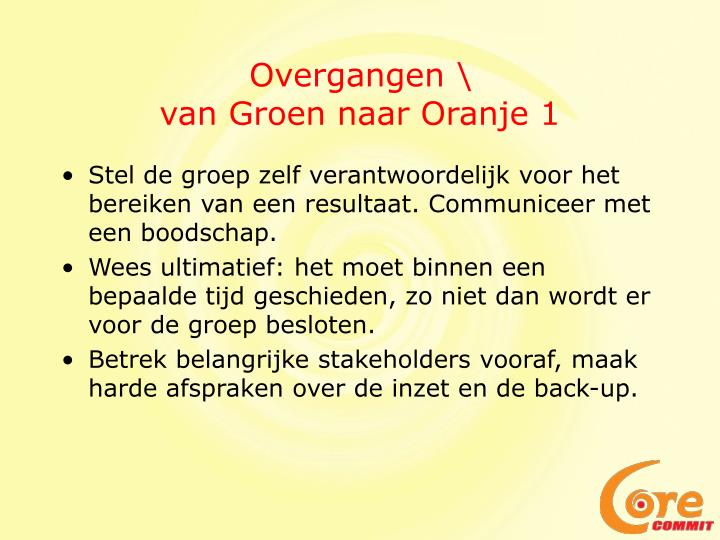The image features a computer-generated text graphic set against a pale yellow, cream-colored swirl background. Prominently displayed at the bottom right-hand corner is the brand logo "Core Commit" in an orange hue with a slight red gradient. The main body of text, which appears to be in Dutch, starts with a large capitalized line in orange: "OVERGANGEN /." Below this in smaller uppercase text is "VAN GROEN NAAR ORANJE 1" in black text, followed by a series of black printed sentences. These sentences appear as bulleted points or paragraphs with details on responsibilities and goals such as setting group accountability and achieving results. The text includes phrases like "STEL DE GROEP ZELF VERANTWOORDELIJK VOOR HET BEREIKEN VAN EEN RESULTAAT" and "COMMUNICEER MET EEN BOODSCHAP." Additional details discuss strategic planning and stakeholder involvement, evident in lines such as "BETREK BELANGRIJKE STAKEHOLDERS VOORAF" and "MAAK HARDEAFSPRAKEN OVER DE INZET EN DE BACK-UP." The dimensions of the image are approximately 8 inches across by 6 inches tall, without any border.